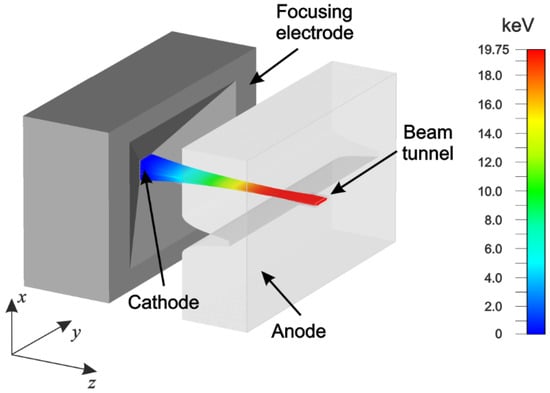The image is a detailed, textbook-quality digital art rendition of a possible electrical device. On the left side, there is a gray rectangular prism labeled "focusing electrode," with arrows pointing from it to the coordinates X, Y, and Z. Adjacent to it is another rectangular object, which is light gray to translucent white and labeled "anode." Emerging from the focusing electrode is a rainbow-colored path marked "cathode," which extends to the end of the diagram where it is labeled "beam tunnel," indicating an opening at a slightly altered right angle of approximately 105 degrees. On the right-hand side of the image, there is a scale gradient ranging from bright red at the top, marked at 19.75, to royal blue at the bottom, marked at 0. The scale is labeled "KEV," suggesting it is a measuring device for energy levels associated with the beam tunnel.